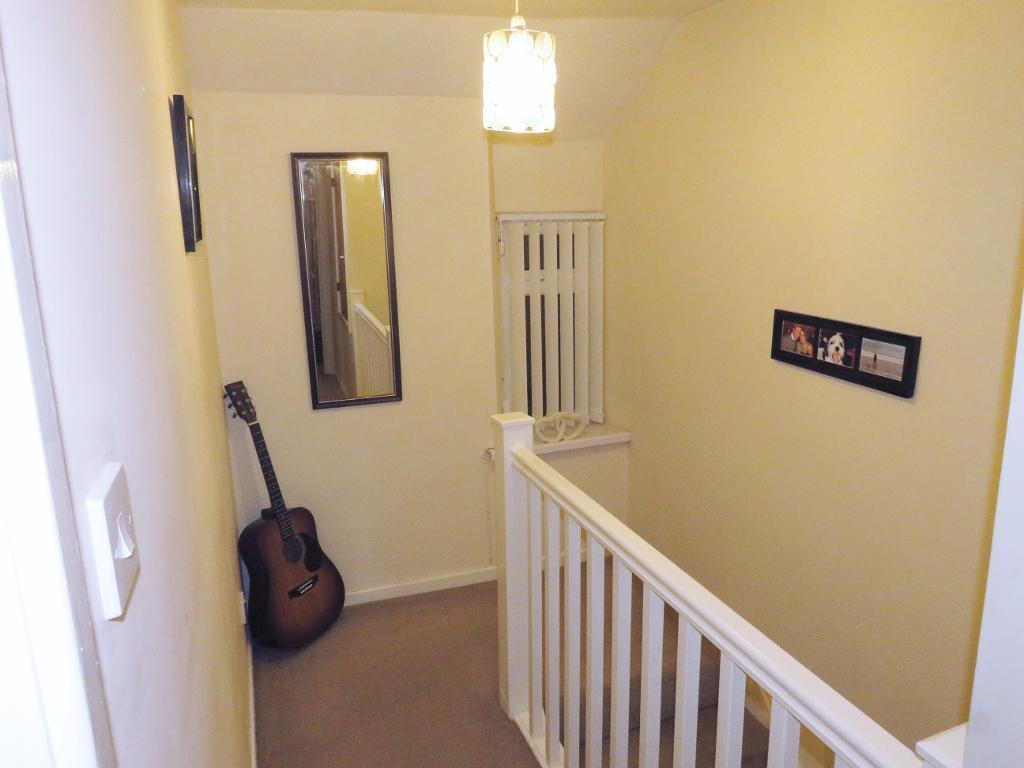The image captures a well-lit upstairs hallway in a house with various objects and features. On the right side of the photo, there is a light yellow or cream-colored wall adorned with a rectangular picture frame containing three smaller images—likely of two people, a dog, and a person by the ocean. Centrally located in the image is a white stair railing with vertical slats, indicating the presence of a staircase leading downwards. The left part of the image shows a white wall where a light switch is visible towards the bottom. In the bottom left corner, a guitar leans against the wall next to another wall, adding an artistic flair to the setting. Just above the guitar, a rectangular mirror with a brown border is also mounted on the wall. The hallway floor is brown, possibly carpeted, adding warmth to the space. In the center-top of the image, a cylindrical-shaped light fixture hangs from the ceiling, illuminated with a yellowish glow, effectively lighting the area. The scene highlights a comfortable and personalized space within a house.